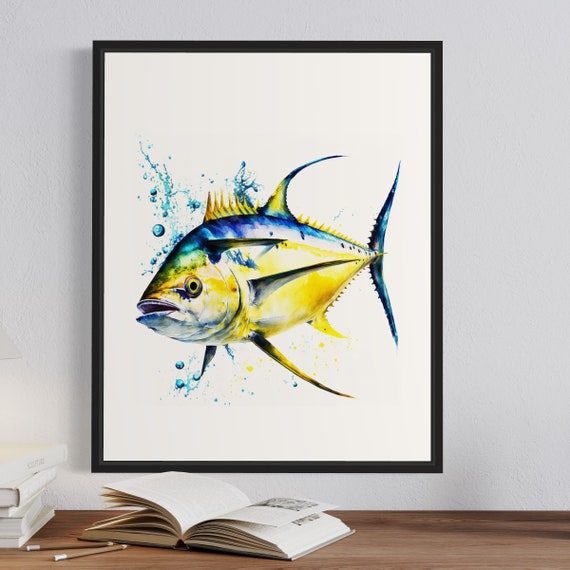This detailed image features a framed drawing or painting of a fish, resembling a tuna. The artwork, enclosed in a black frame and set against a light gray (or lilac gray) wall, showcases a fish with a predominantly yellow or gold body with touches of white and blue. The upper part of the fish and its fins exhibit shades of blue and dark blue, while its tail is depicted in dark blue. The fish is illustrated at a three-quarters angle, showing its face and one side. Notable features include its ridged spikes along the spine and lower back, a partially open mouth, and a circular eye with a black center and gold rim. The fish is depicted splashing in water, which includes gold and blue splashes and bubbles emerging from its head.

Below the framed image is a brown desk. On the desk, right beneath the picture, lies an open book, roughly halfway through. To the left of the open book are two brown pencil-like utensils, and further left, nearly cut out of the frame, is a small stack of three or four white-colored books. The background of the fish painting is white, enhancing the contrast and vividness of the fish's colors against the simplicity of the frame and the surrounding wall.